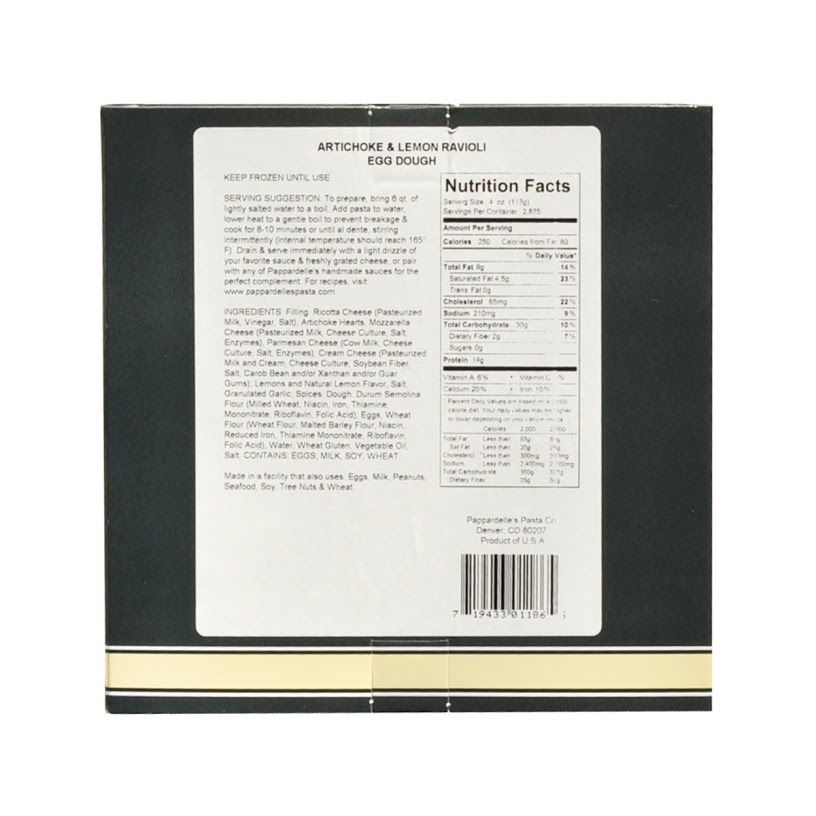This image features the back of a nutrition label for a product named "Artichoke and Lemon Ravioli Egg Dough," clearly labeled at the top in bold black text. The label advises consumers to "Keep Frozen Until Use" and includes a serving suggestion, though the print becomes illegibly small beyond this point. Below these instructions, the ingredients list is provided. Additionally, there is an allergy warning at the bottom, stating that the facility processes egg, milk, and peanuts. A barcode is situated at the very bottom, next to a "Product of USA" note. The nutrition box, which is rectangular and in classic black and white, details critical nutritional information such as serving size, calorie count, and various other dietary specifications.